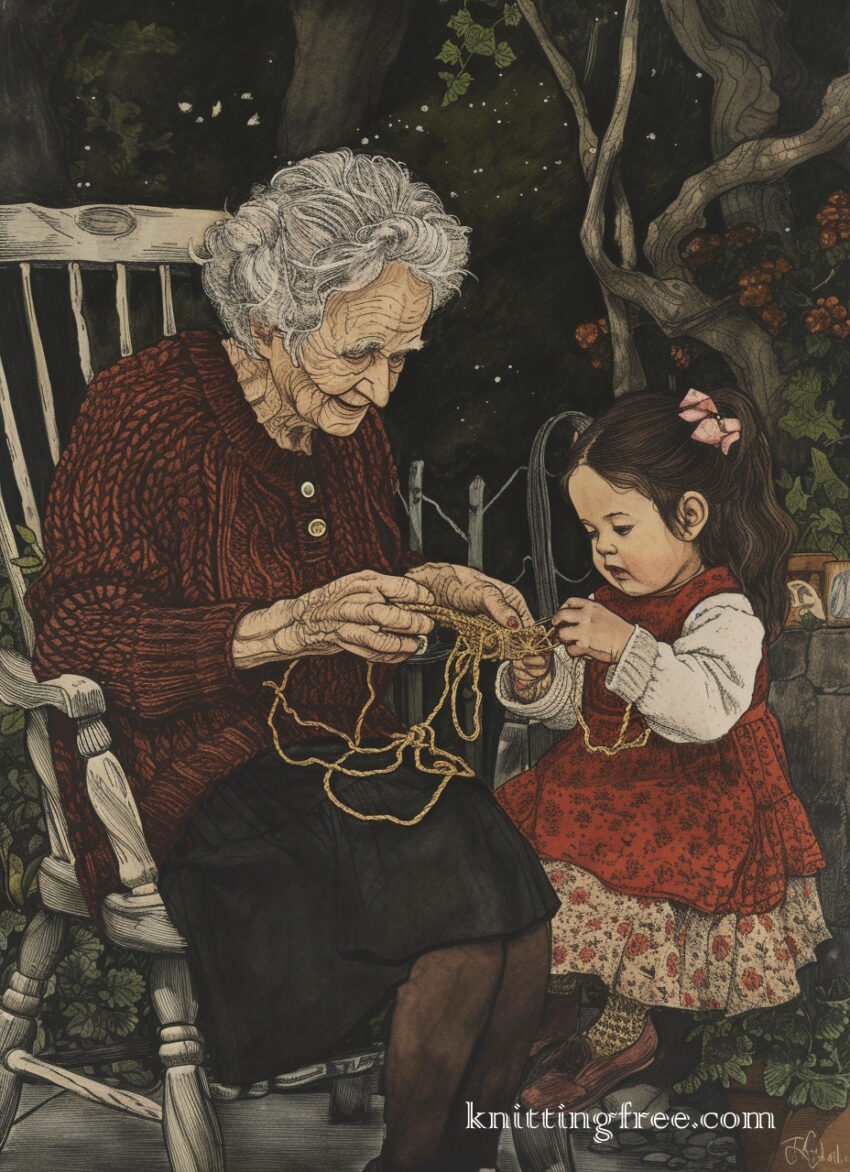The image is an illustration of an elderly woman and her granddaughter sitting together outside on a front porch at nighttime. The sky is dark, studded with a myriad of stars shining through. Behind them, twisted brown tree branches frame the serene scene. The elderly woman, with very wrinkled beige skin and short gray hair, is adorned in a burgundy knit sweater and black skirt. She sits in a light-colored wooden rocking chair. Beside her is her granddaughter, a young girl with brown curly pigtails tied with pink bows. The girl is dressed in a white layered dress embellished with pink flowers, complemented by a red apron and a little white shirt underneath. Her outfit is completed with pink shoes. Both characters are intently knitting with beige-colored yarn. The serene, evocative ambiance suggests a timeless quality, possibly reminiscent of an era gone by. In the bottom right corner of the painting, "knittingfree.com" is inscribed in white letters along with the artist's signature.